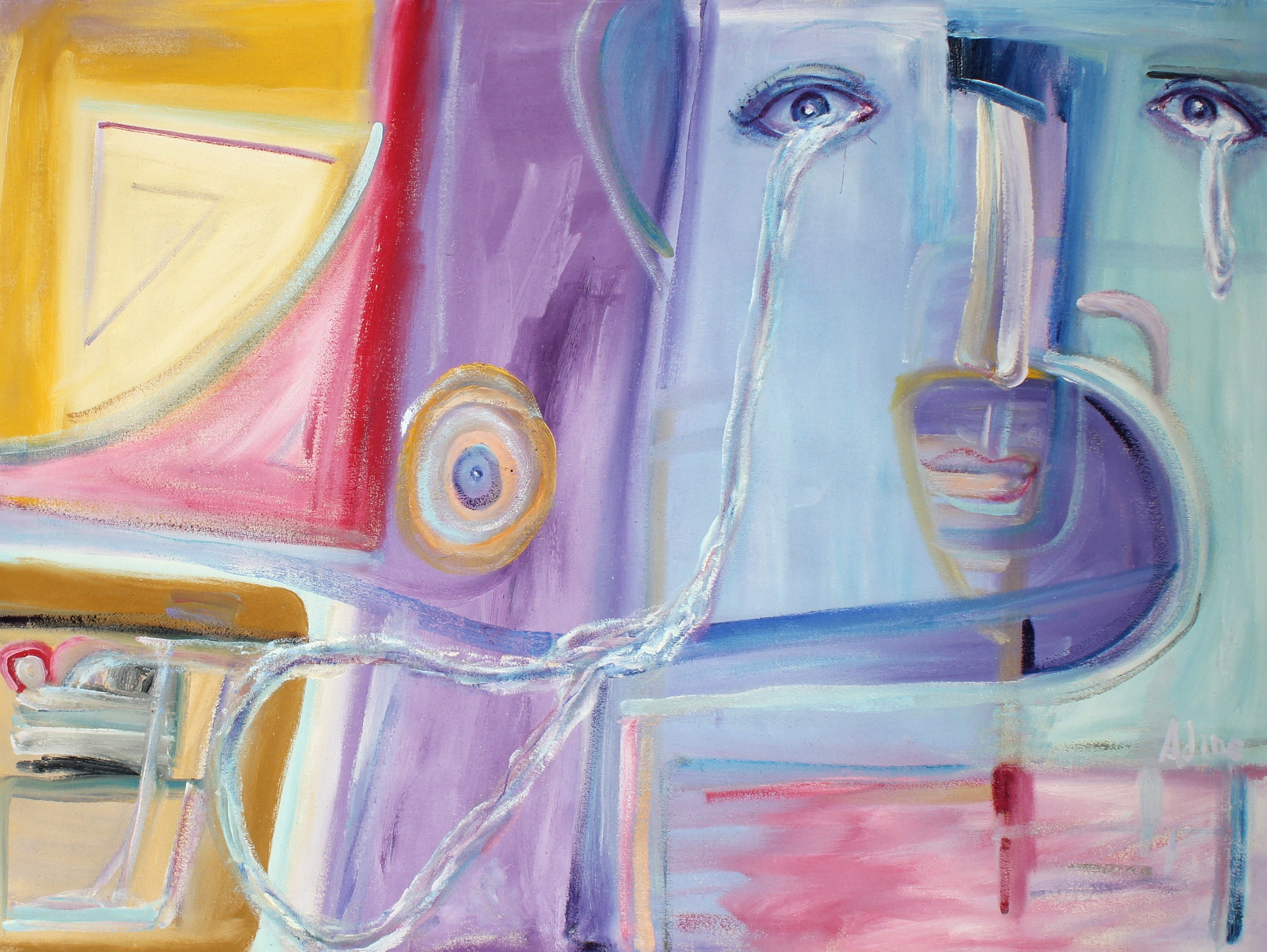The image is a rectangular abstract painting, approximately six inches wide and four inches high. Dominating the upper right corner is a pair of eyes with their outer corners slightly sloped downward; the right eye is set against a green background, while the left eye has a light purplish hue behind it, making it appear to gaze rightward as the white area in front gives an impression of a nose. Each eye is depicted with tears streaming down, with the left eye's tear forming a blue line that curves and circles towards the lower left corner of the artwork.

In the lower right corner, there is a box filled with pink paint, intersected down the center by a purplish-pink band adorned with yellow and white circles with blue centers. The upper left corner showcases a square with a red lower right section and a yellow upper left section. Meanwhile, the lower left corner contains a dark mustard-yellow box featuring a lighter center that depicts what resembles a light blue car.

The painting is filled with a vibrant palette, including shades of yellow, pink, red, purple, lilac, blue, teal, seafoam green, and deeper brownish yellows. These colors, along with the various shapes and forms, contribute to the abstract, almost surreal, nature of the piece, reminiscent of Picasso’s work. The overall setting gives an impression of a whimsical piece of wall art.